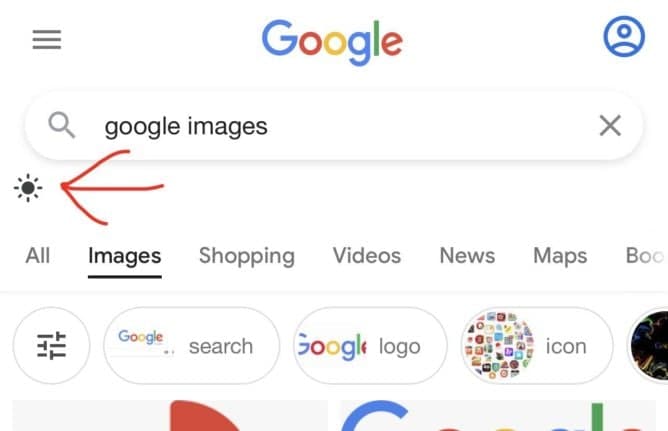The image depicts a partial screenshot of a Google search results page with a white background. Dominating the center is the prominent Google logo: both 'G's are blue, the first 'O' and the 'E' are red, the second 'O' is yellow, and the 'L' is green. At the top right corner, a blue circular icon with a generic user profile is visible. Below this, the search bar shows the text "Google images".

To the left beneath the search bar, there is a hand-drawn red arrow pointing to an image of a sun. Arrayed below are various tab options. The options include: "All," "Images," "Shopping," "Videos," "News," "Maps," and a tab partially cut off ending with "BOO." The "Images" tab is underlined, indicating it is the active selection.

Underneath these tabs, there's an icon: a circle with embedded lines, suggesting some form of graphical representation. Following this, there are more tabs including: "Google search," "Google logo," and "icon." The corresponding image beside the "icon" tab is a circle filled with numerous, indistinct mini-icons, which are blurred and difficult to identify. Additionally, on the far right is the partial view of another circle with a dark background, containing indistinguishable content. The page abruptly cuts off, partially displaying the word "Google" once more before the visible section ends.